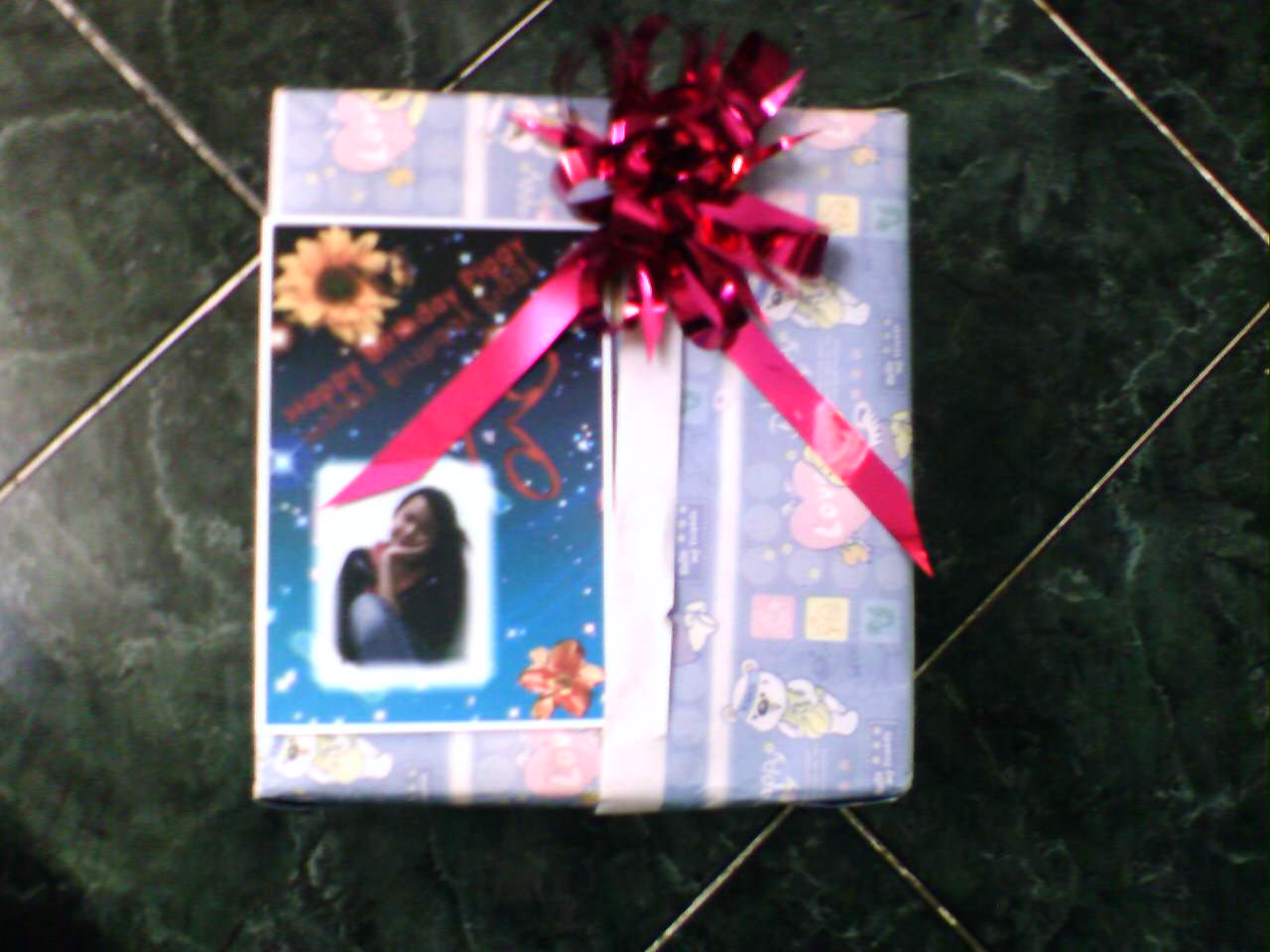The photograph captures a neatly wrapped, square-shaped present placed on a dark green, square marble floor. The gift is adorned with light lavender wrapping paper featuring playful, baby-themed designs, including hearts with the word "love," and white bear illustrations. A white ribbon secures the wrapping, with a prominent magenta bow fixed at the top center, adding a bright, eye-catching contrast. On top of the present, a card reads "Happy Birthday Piggy," though the sender's identity remains unknown. The image also depicts a white banner running vertically across the package, and a small, outlined square featuring a woman resting her head sideways in the palm of her hand. The scene is completed with the presence of a shiny, metallic red bow tie integrated into the decorative elements of the gift.